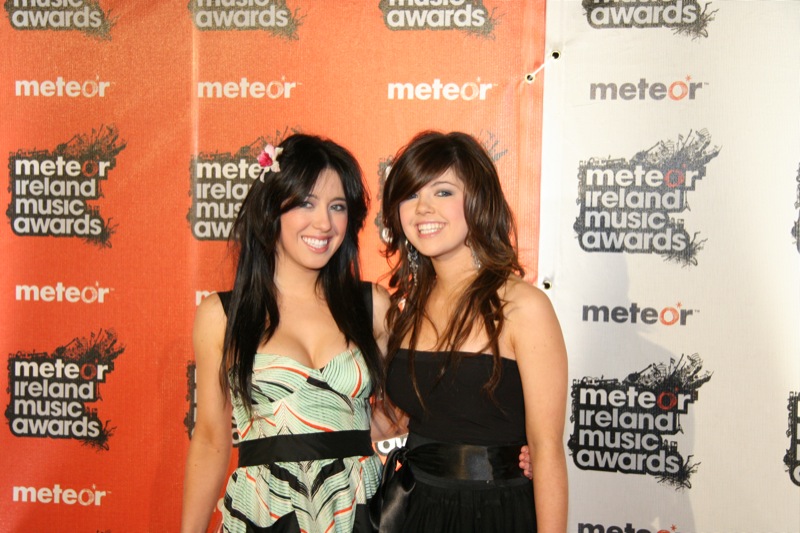In this vibrant image, we see two young girls gleefully standing in front of a promotional banner for the Meteor Ireland Music Awards sponsored by Meteor. Both girls have big smiles with their teeth showing, and their lively eyes exude excitement. They are dressed in stylish, low-cut dresses; the girl on the left wears a striking green dress with black straps, complemented by a flower in her long black hair. The girl on the right dons an elegant black dress, her long brown hair framing her face. Each girl accentuates her dress with a belt. Their fuzzy hair adds a playful touch to their appearance. Behind them, the background features several banners in various colors: prominently three in orange, and others in white, blue, and green.